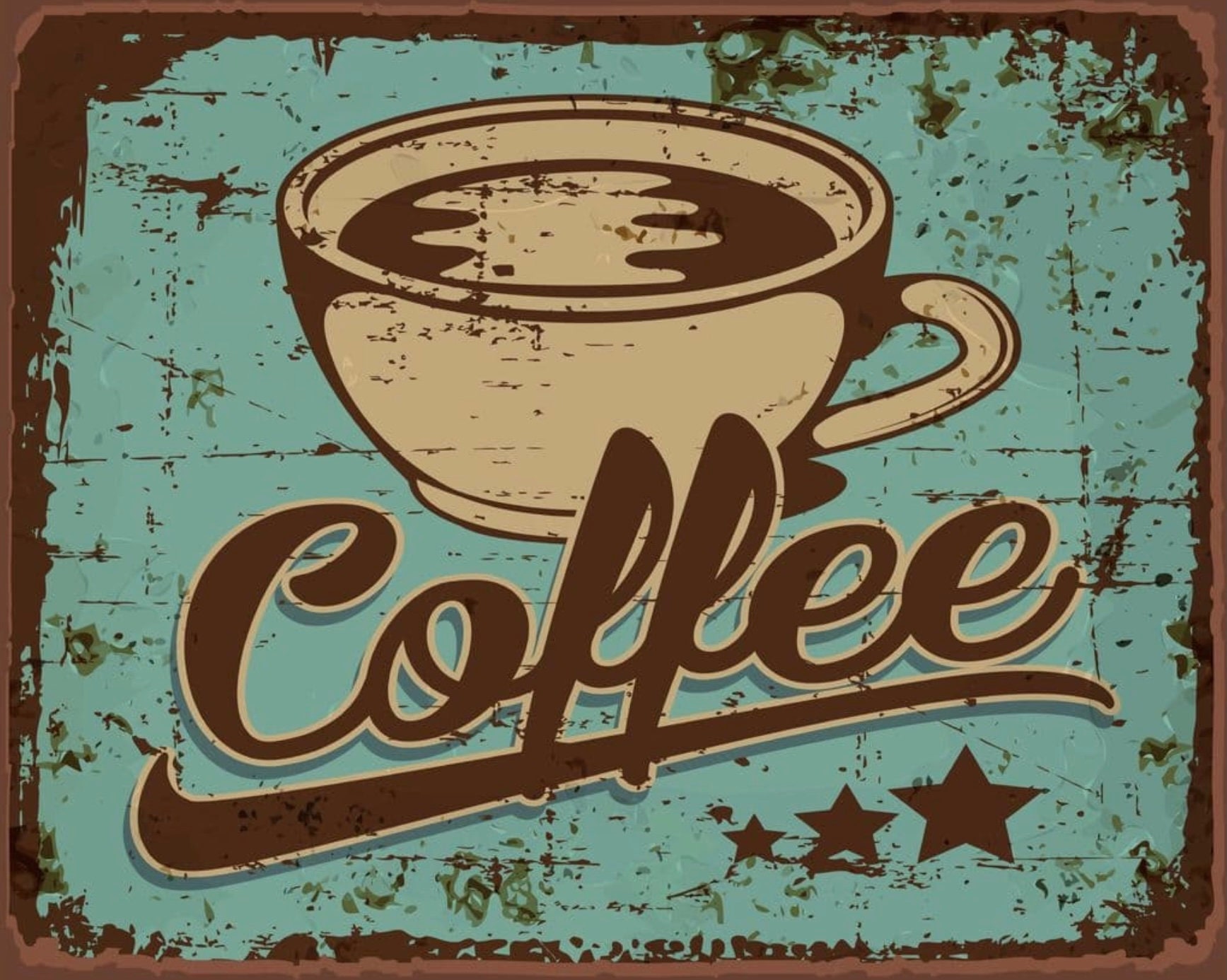This image depicts a vintage, rustic sign for a coffee shop, roughly three feet tall by three feet wide. The sign has a weathered, distressed appearance, featuring rusty metal edges and an aqua blue background with patches where the rust is visible. At the center is a large, stylized white coffee cup with brown shading to define its shape. The cup appears slightly worn, adding to the sign's antique charm. Above the cup, the word "Coffee" is prominently displayed in dark brown cursive letters, outlined in white to make it pop against the backdrop. Below the word, there is a brown stripe also outlined in white, and beneath this stripe are three stars of varying sizes, arranged in a row. This sign, reminiscent of old cafe or diner advertisements, exudes a collectible, decorative appeal perfect for a cozy kitchen setting.